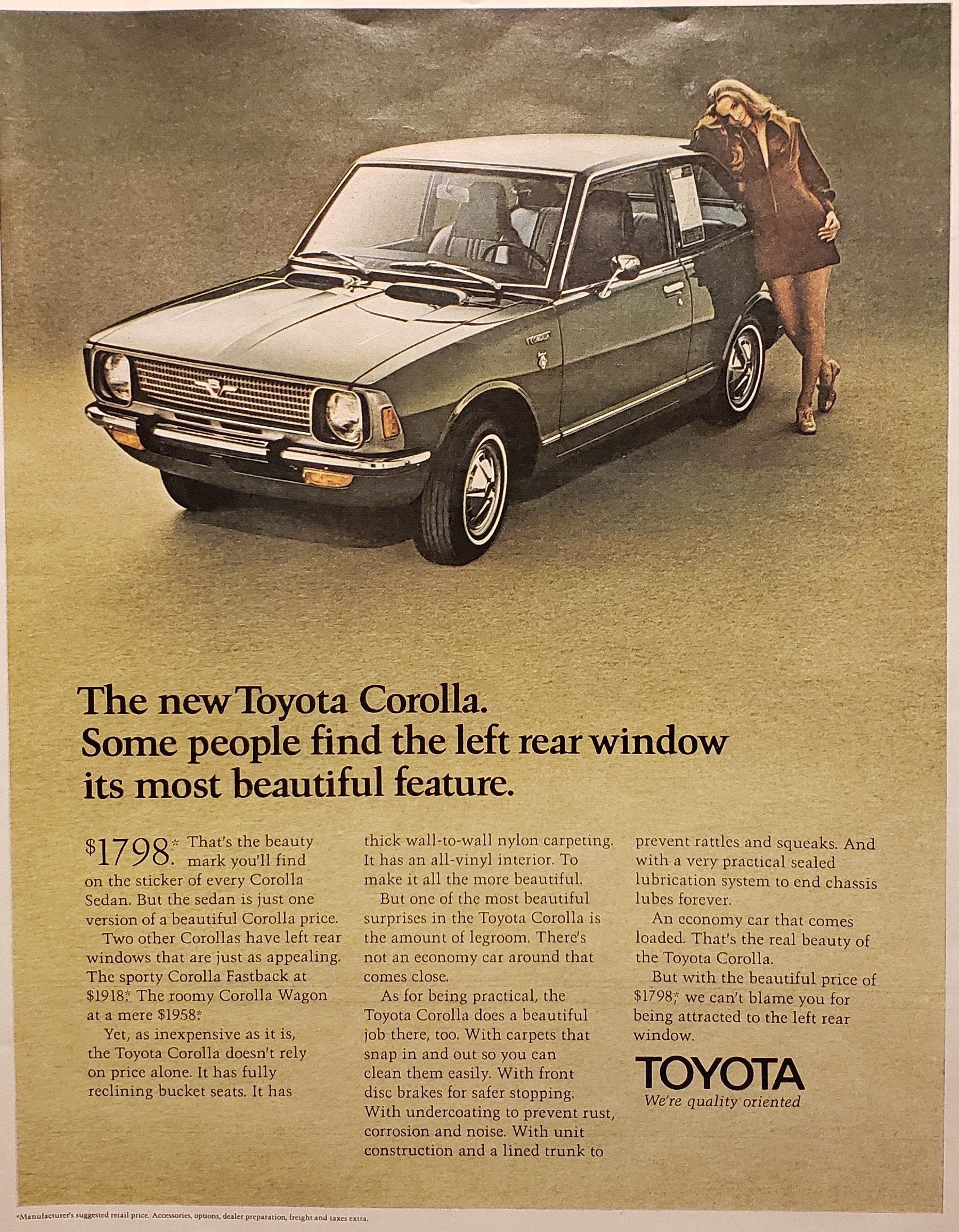This is a vintage advertisement for a new Toyota Corolla, most likely from the 60s, 70s, or 80s, characterized by its sepia-toned, gray, and brown color palette. The background features a gradient that transitions from dark brown at the top to a light tan or sandy color at the bottom. Dominating the top half of the ad is the image of a tan-colored Corolla, described by some as a greenish-brown or army green. The car, which looks fairly basic with chrome trim, is angled slightly towards the viewer and to the left.

Leaning against the left rear window of the sedan is a woman dressed in a brown miniskirt dress with a zipper detail, suggesting fashion cues from the 60s. Her curly, blonde hair (sometimes described as long and brown) cascades down as she adopts a confident pose, with one hand on her hip and her legs crossed at the ankles.

Bold text below the image reads, "The New Toyota Corolla. Some people find the left rear window its most beautiful feature." Alongside this, the remarkably affordable price of $1,798 is prominently displayed. Further text in the lower half of the ad extolls the virtues of the Corolla, discussing its features in detail. In the bottom right corner, the Toyota logo is featured with the tagline, "We’re quality oriented," underscoring the brand’s commitment to quality craftsmanship.